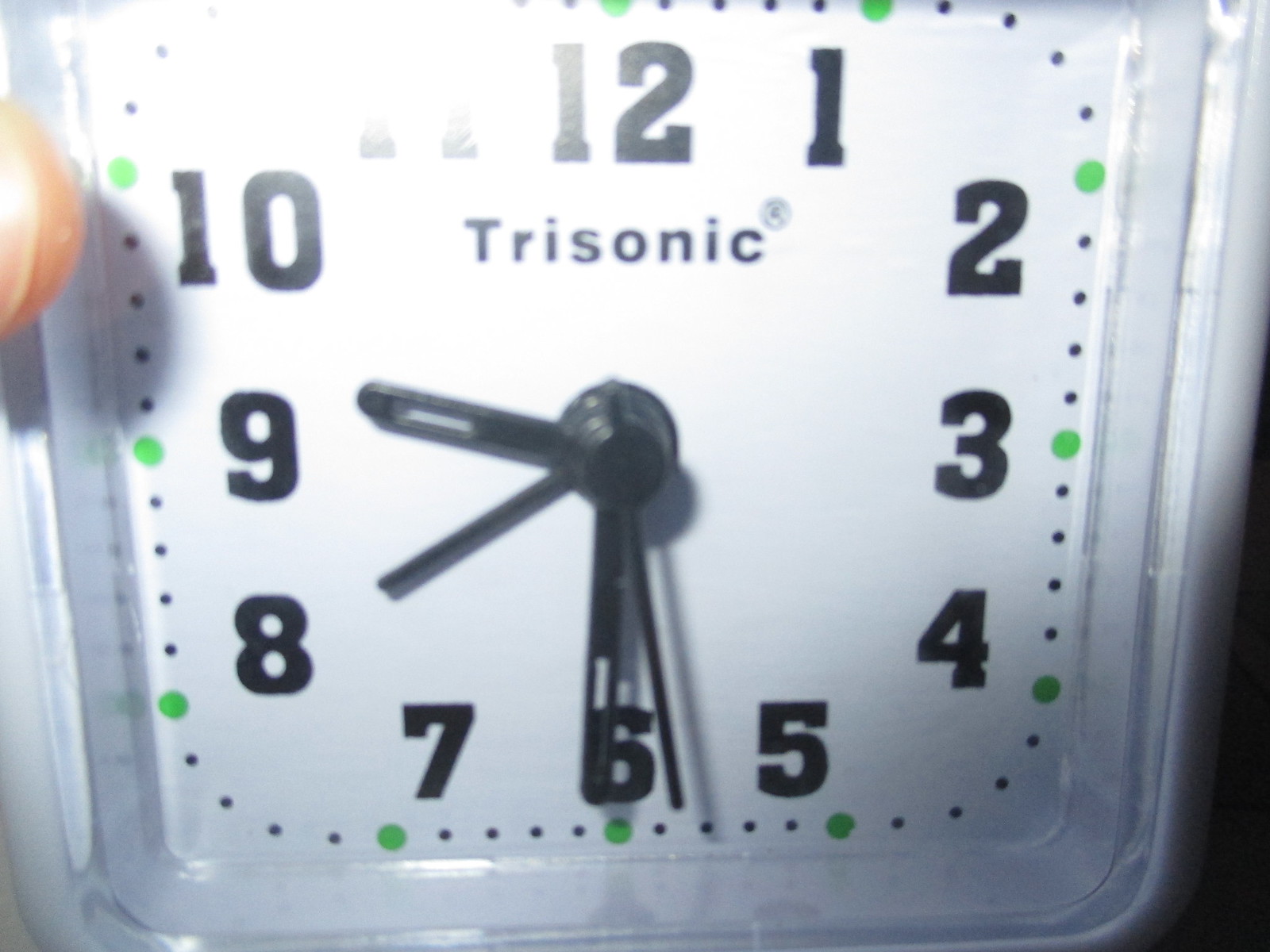The highly zoomed-in image showcases a square-shaped clock. The clock features a gray frame with bold black numbers clearly displayed in a clockwise manner: 12, 1, 2, and 3 on the right; 4, 5, and 6 at the bottom; 7, 8, and 9 on the left, ascending to 10 and 11. The brand name "Trisonic," printed in black text, is prominently visible. The minute hand is positioned at the 6, while a shorter hour hand points just past the 9, and another shorter hand is near the 8. The second hand is captured mid-motion, situated between the 6 and 5 marks. A thumb, casting a grayish shadow, enters from the left side of the image, holding the clock. The bottom right corner of the image subtly reveals a dark background.